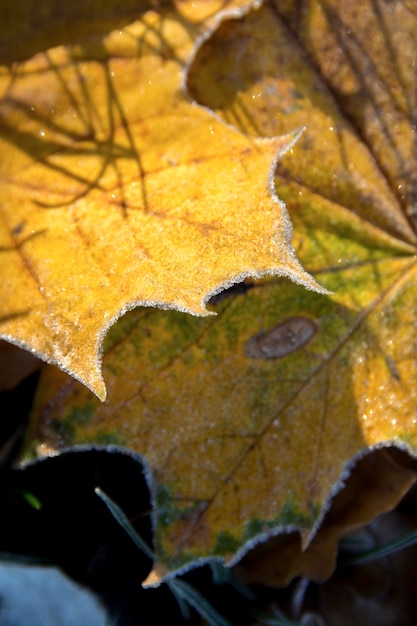In this close-up, vertical photo, we see a cluster of overlapping leaves in the process of changing colors, indicative of a fall day. Dominating the scene, a bright yellow-orange leaf with a silverish trim takes center stage in the top left, bathed in sunlight and sharply detailed with dark orange veins. This prominent leaf faces right, standing out vividly against the darker, shaded background.

Beneath this sunlit leaf lies a larger yet hidden leaf, extending from the top right to the bottom left of the image. Despite its sprawling presence, this leaf remains in the shadows, displaying a blend of yellow, orange, and green hues with darker gray and brown spots in its center.

The bottom third of the image fades into a dark, almost black, indistinct foreground, accentuating the detailed leaves above. The leaves' jagged edges add to the texture, highlighting their transitioning state and the intricate play of light and shadow within the composition.